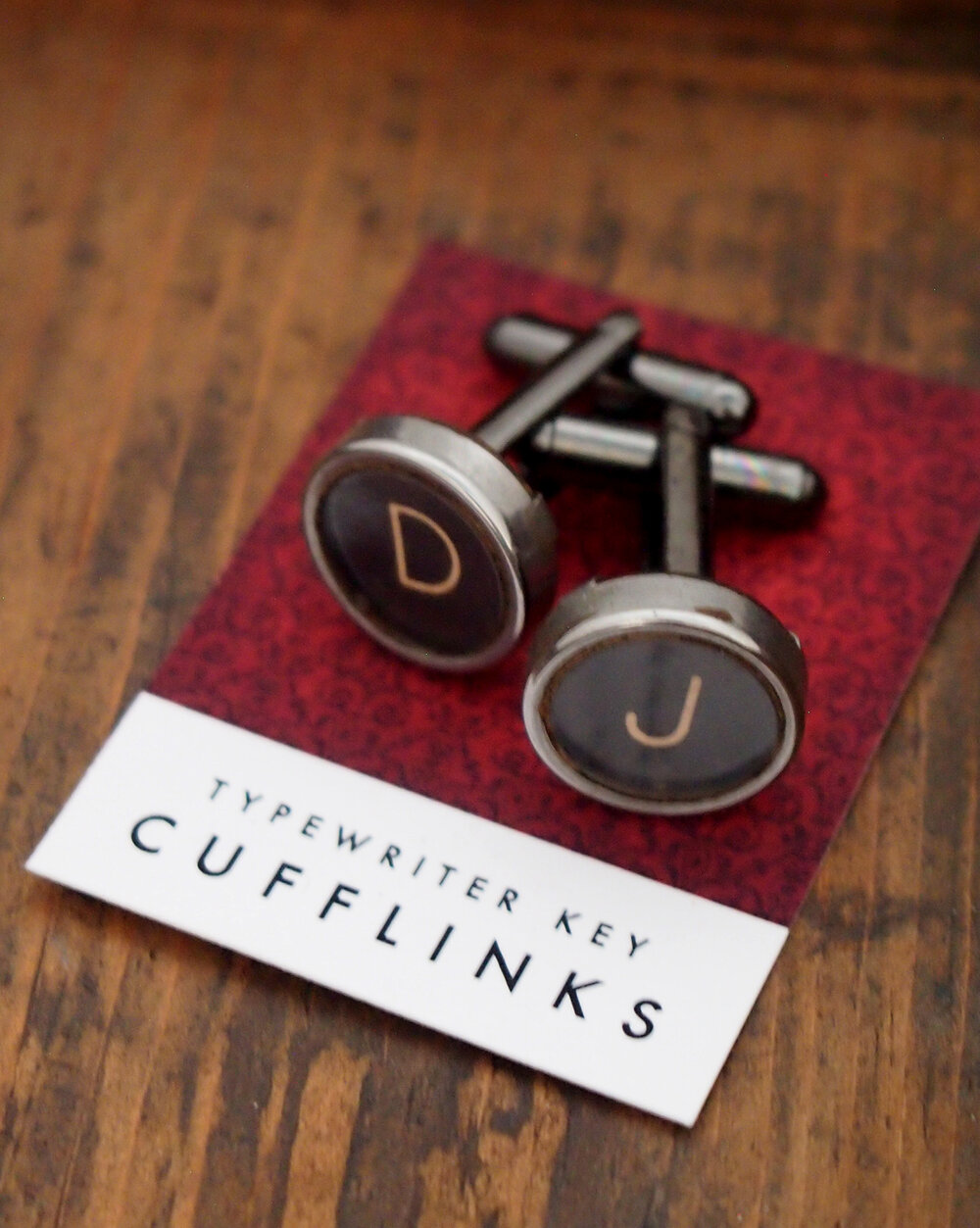This photograph showcases a pair of typewriter key cufflinks, displayed on a red card with a black pattern, possibly paisley. The cufflinks, featuring the letters D and J in white text on a black background, are crafted from a darker metal that resembles blackened silver. The card itself bears the text "typewriter key cufflinks" in black over a white rectangle at its base. The card is placed on a light brown wooden surface, adding a rustic touch to the professionally taken, clean and minimalistic product shot.